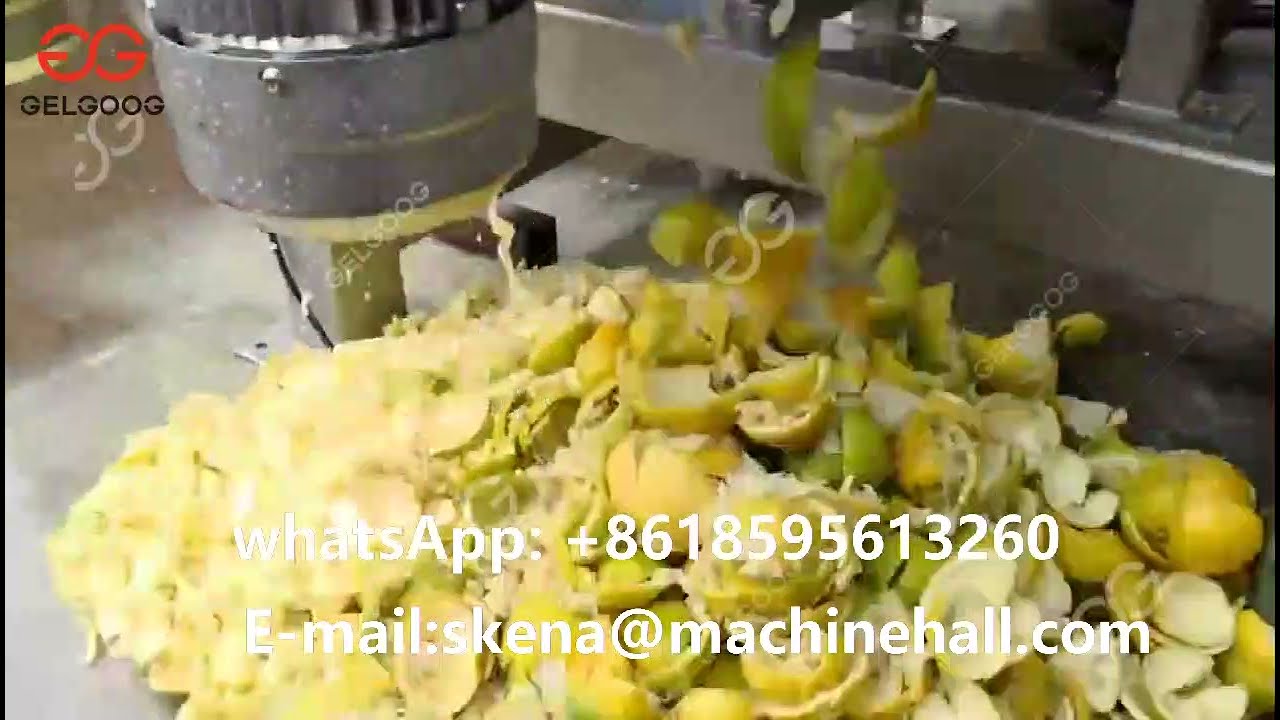The image depicts a close-up of several fruit parts scattered on the floor, primarily in shades of yellow, orange, and green, suggesting they are likely segments of lemons, oranges, or limes. These fruits appear to have undergone processing, possibly in a juice extractor, evidenced by the pile of rinds collected below the machine. On the left and towards the top right of the image, parts of a metallic machine are visible, including a round, bucket-like container and a metal bar. The top left corner features a prominent logo with red overlapping Gs, labeled "Gelgoog," along with a faded white version of the same logo underneath. Text on the image provides contact information: "WhatsApp +861-8595-6132-60" and "email skena@machinehall.com," indicating potential customer service or product details. The scene is indicative of a commercial fruit processing operation.